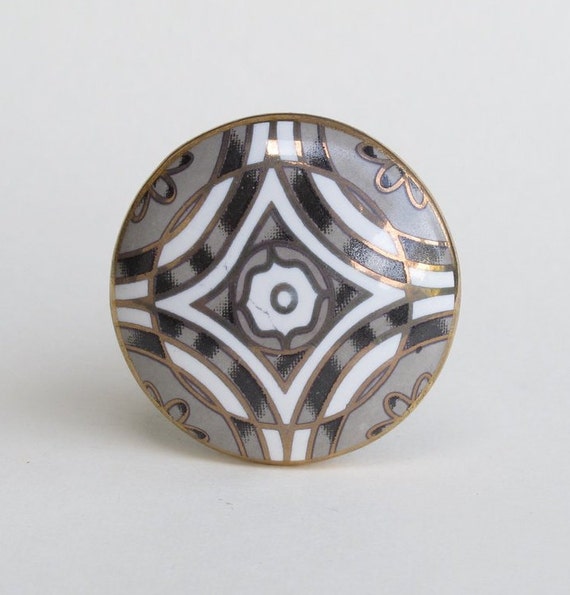This perfectly square photograph showcases a meticulously detailed round object, possibly a piece of jewelry like an earring, brooch, or button, set against a plain gray background with a soft shadow cast to the left, indicating the light source from the top right. The object features an intricate and artistic design, with a prominent gold trim encircling its circumference. Inside this outer gold border, there is a series of alternating gold, white, and gray sections forming a geometric pattern that resembles a flower or star shape. The very center of the piece is composed of concentric rings: a black circle enveloped by a white circle, followed by another gray and finally a white center. The overall design incorporates elements of both circular and flower-like motifs with no text present, focusing solely on the elaborate and eye-catching craftsmanship of the object.